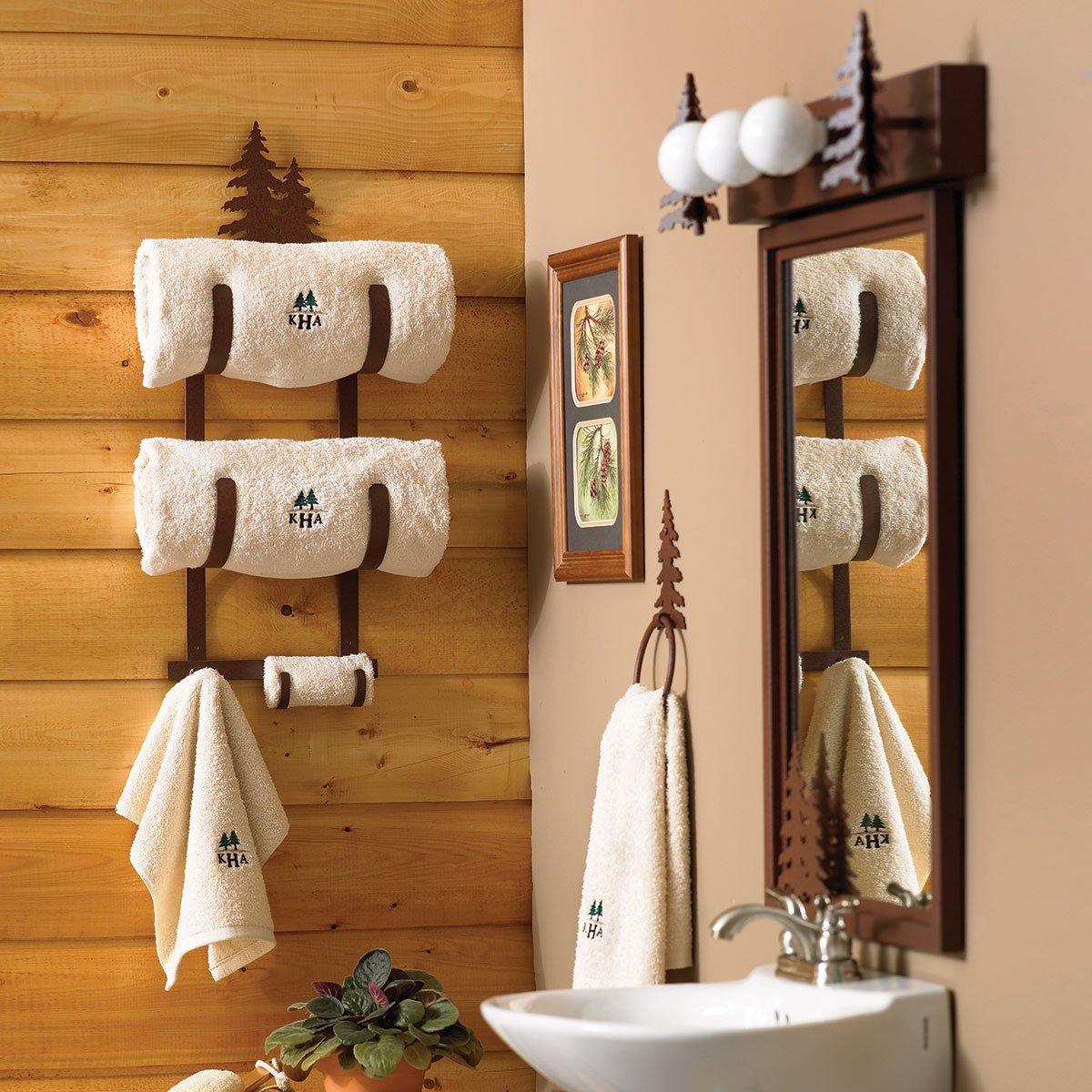This image captures a well-maintained bathroom corner with distinct wood and metal accents. The left wall features horizontal brown wooden planks, holding a brown metal rack adorned with pine tree silhouettes. This rack functions as a towel holder with three hooks: the top two holding large white towels, the middle one a smaller white wash rag, and the last just a hanging towel. All towels are embroidered with "KHA" and green tree symbols. The right wall is a light brown painted surface, embellished with a framed photo of greenery and a large mirror, both encased in wooden frames. Above the mirror, a wooden light fixture with three white globe bulbs extends the rustic theme. Another green metal hook shaped like a pine tree holds an additional white towel. Below the mirror, a white sink sits with a silver faucet. Overall, the bathroom exhibits a clean, cohesive decor with meticulous wood and tree-themed details, suggesting it might belong to a hotel or a specially curated interior.